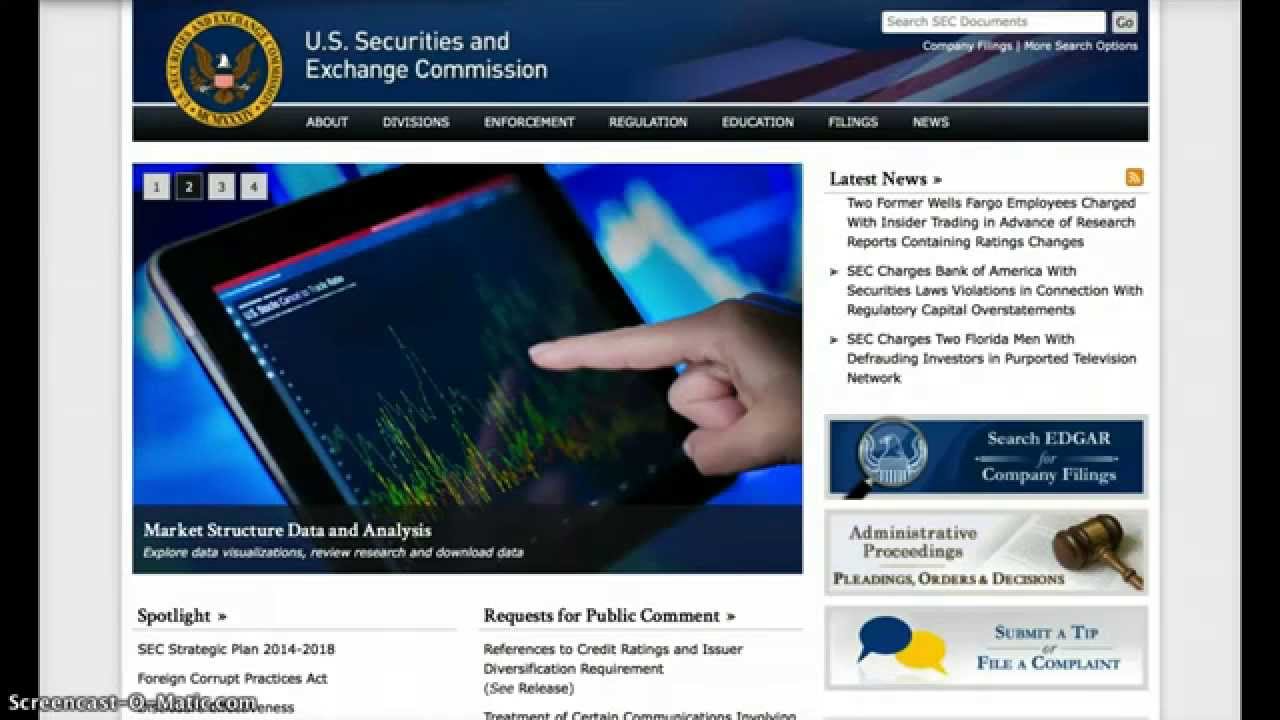The image showcases the homepage of the U.S. Securities and Exchange Commission website. On the left, a prominent gold ring features a dark brown wing logo centered within it, accompanied by white text. The top right corner hosts a search bar with a gray "Go" button. The website's upper section has a black and dark blue background, transitioning to a solid black background below. 

Displayed from left to right are the main categories: About, Divisions, Enforcement, Regulation, Education, Filings, and News. Beneath these categories, an image depicts a person using a touch screen device to display a chart, with text below reading "Market Secure, Market Structure, Data and Analysis."

On the right side, the "Latest News" section with a white background highlights three clickable articles. Below this section, a dark blue design invites users to "Search Edgar," followed by a section on "Administrative Proceedings" featuring a court gavel on a light gray background. Further down are options to "Submit a Tip," "File a Complaint," indicated by a dark blue message icon and a yellow message icon, on a light gray background.

The bottom left shows a "Spotlight" section with three articles and a "Request for Public Comment" area, featuring two clickable options. The overall page design includes light gray backgrounds on the left and right, transitioning to black on the very outer edges.